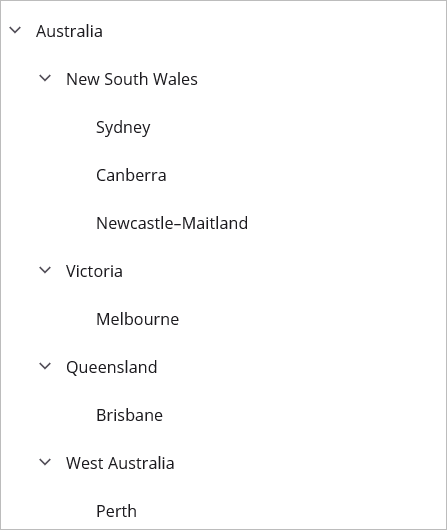A neatly organized list of places is presented on a white background, divided into distinct categories by thin black lines that form the outer perimeter of the box. The lines are noticeably thinner than the text inside, emphasizing the boundary of the listed content. In the upper left-hand corner, the first category marked by a downward arrow is "Australia." Underneath "Australia," another downward arrow points to "New South Wales," indicating it as a subcategory. Within "New South Wales," the list further narrows down to specific locations: "Sydney," "Canberra," and "Newcastle-Maitland."

Proceeding further, the category "Victoria" appears next, also marked by a downward arrow, and leads to the location "Melbourne." Subsequently, "Queensland" is listed with a downward arrow directing to "Brisbane," followed by "West Australia" leading to "Perth." Each category and its corresponding location are logically arranged, highlighting the hierarchical structure from country to states, then to their respective cities. This clear and systematic arrangement makes it easy to understand that Sydney, Canberra, and Newcastle-Maitland are part of New South Wales; Melbourne is in Victoria; Brisbane is in Queensland; and Perth is in West Australia, all within the broader category of Australia.